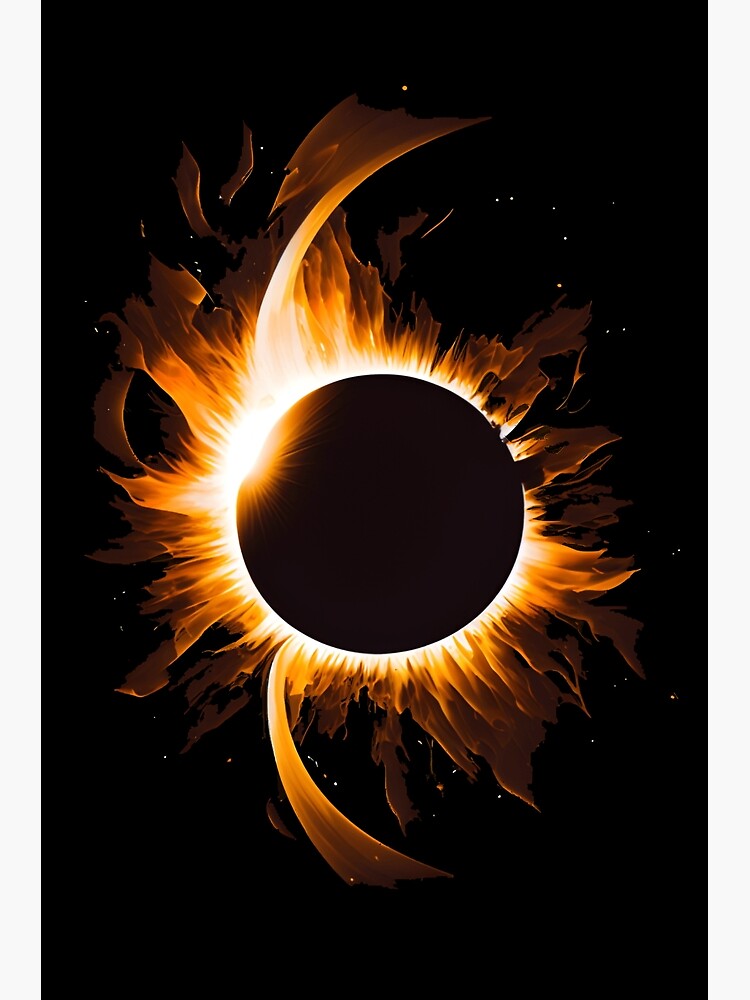This digital painting vividly portrays a solar eclipse against a black space backdrop peppered with white and yellowish-orange stars. At the image's core is a pitch-black circle, surrounded by brilliant light radiating outward. The light transitions from white at the edges to intense orange further out, reminiscent of the sun's rays. Particularly striking are the artistic, curved solar flares or flames that arch majestically around the circle, with two dominant ones extending further to the top-left and bottom-right. Additionally, a partial sunspot is visible at the top-left, contributing to the realistic yet stylized depiction of this celestial event.